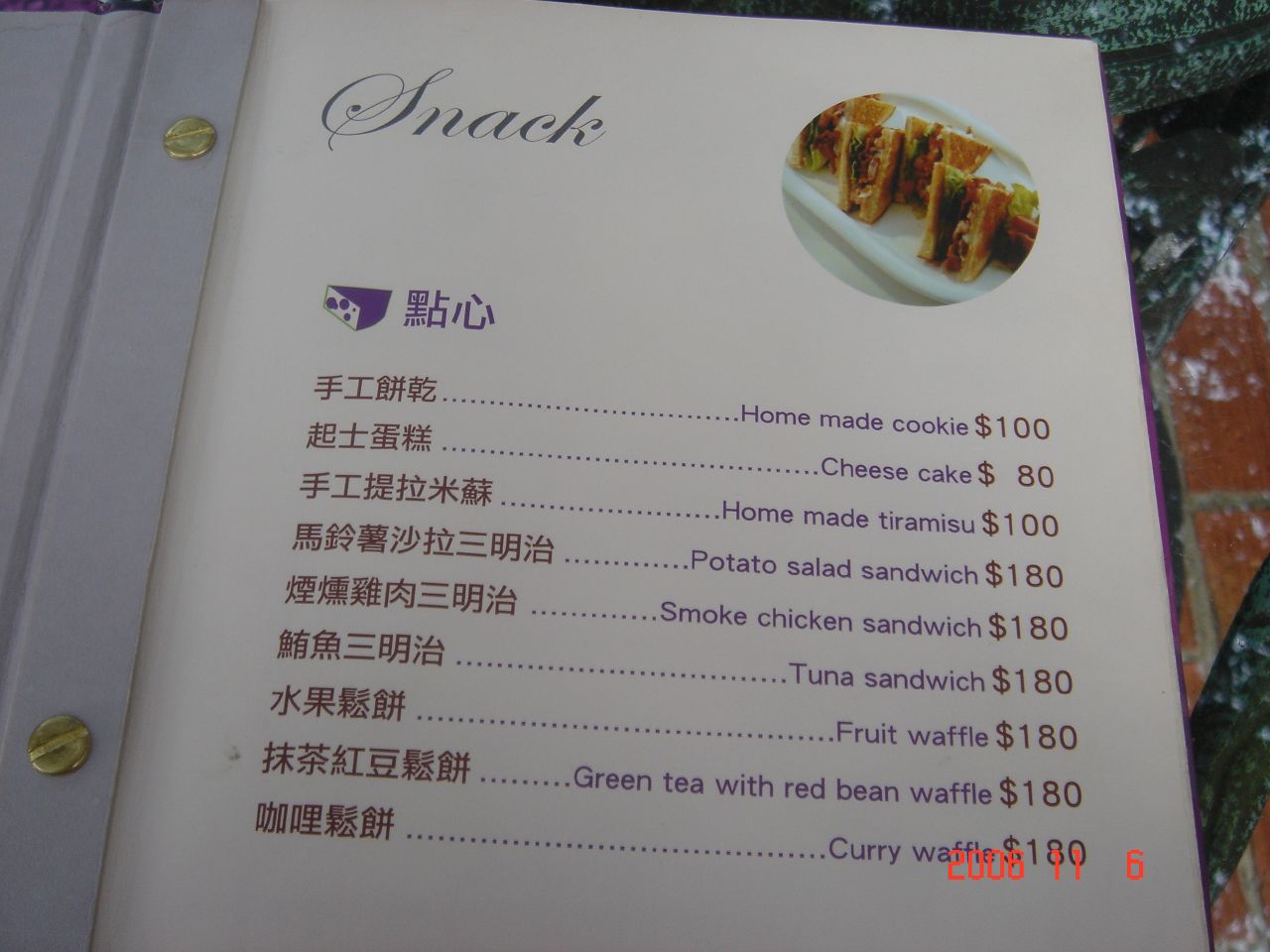This color photograph showcases a section of an elegantly bound menu, placed upon a vibrant and intricate tablecloth. The tablecloth displays a refined pattern of greens, pinks, and blues, crafted from beautiful fabric, suggesting a sophisticated dining atmosphere. 

The menu is open to a page labeled "Snack" at the top, written in yellow and gray script. The page itself is a very light grayish lavender, adding to its elegant appearance. A round photograph is featured on the menu page, depicting hors d'oeuvres, including small, triangle-shaped sandwiches, hinting at the refined culinary offerings. 

The menu items are presented in two languages: Chinese or Japanese on the left, and English on the right. The English menu lists the following delectable items: homemade cookie, cheesecake, homemade tiramisu, potato salad sandwich, smoked chicken sandwich, tuna sandwich, fruit waffle, green tea with red bean waffle, and curry waffles.